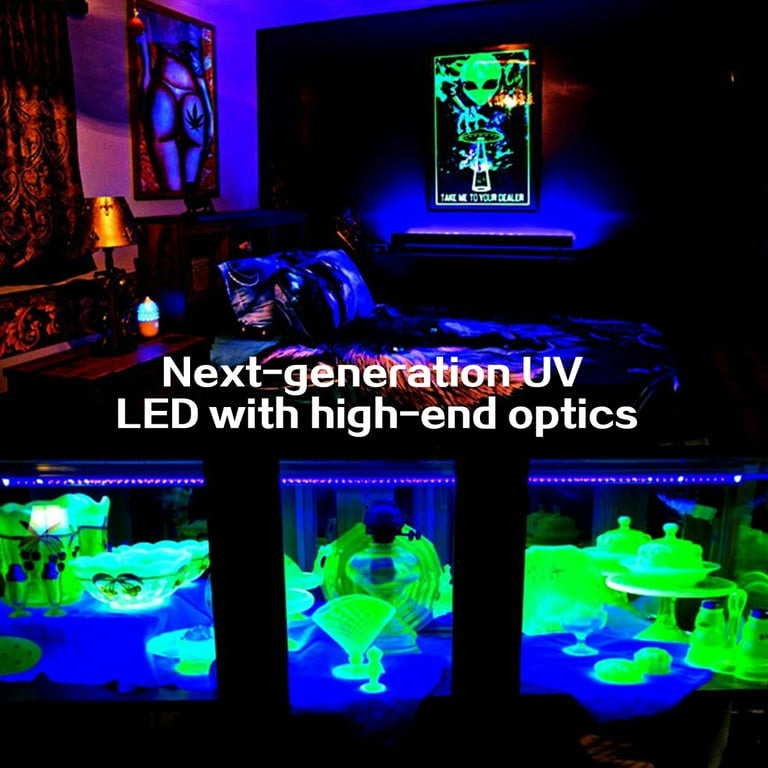The image depicts a dark bedroom bathed in the ethereal glow of UV lights and black lights, creating a surreal and vibrant atmosphere. Centered in the room is a bed with two pillows and a blanket that appear luminescent in shades of blue, purple, and orange due to the UV lighting. Above the bed, the walls are adorned with eye-catching, glow-in-the-dark posters. To the right, there's a poster featuring a green alien and a spaceship with the humorous caption "Take me to your dealer" glowing in bright neon green. Directly above the head of the bed is another poster showcasing a woman's behind with a marijuana leaf tattoo, which also radiates under the UV light.

To the left of the bed, a small wooden bedside table holds a gold lamp and an intriguing, glowing acorn-shaped object in orange and blue. The room is complemented by some brownish curtains visible in the upper left corner. In the middle of the image, striking white text reads, "Next Generation UV LED with High-End Optics," highlighting the advanced lighting technology on display.

The bottom section of the image features a collection of uranium glass dinnerware, including dishes, bowls, cups, and cake holders, glowing intensely in green under the black lights. Surrounding these items are LED strips, adding to the vibrant luminosity of the scene. The detailed arrangement and radiant colors create a visually captivating and somewhat otherworldly experience.